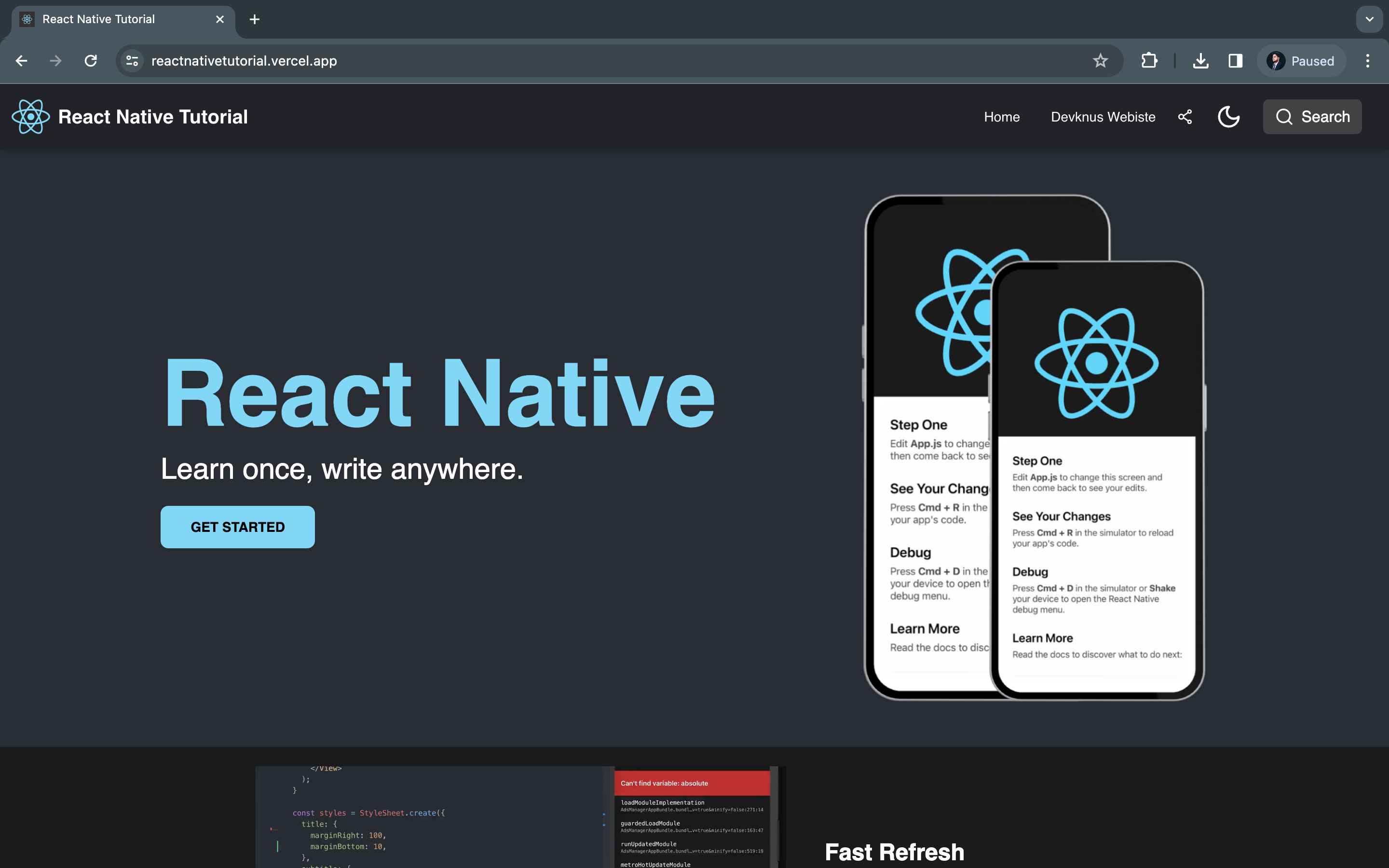**Caption:**

The image depicts a web browser window on a desktop, focused on a tutorial for React Native. In the top-left corner, the title "react-native-tutorial" is displayed, accompanied by a distinctive icon on the right side. The icon features three intersecting blue ovals forming a star shape, with a blue dot at the center.

On the top-right of the browser, there are several tabs labeled "home," "dev," "NAS website," along with icons for share, dark mode, and a grey search button.

Centered on the left side of the page, there is a prominent heading stating "React Native - Learn Once, Write Anywhere." The phrase "React Native" is in blue, while "Learn Once, Write Anywhere" is in white. Below this text, a blue button with black text reads "Get Started," with a dark blue background enhancing its visibility.

To the right, the screen showcases two smartphone interfaces. The background phone is larger, and the foreground phone is smaller, but both display identical content. At the top of the smartphone interface, a blue logo appears against a black background. Beneath the logo, the text is in black on a white background, conveying the following instructions:

- Step 1: Edit `App.js` to change the screen, then return to see your edits.
- To see changes, press Command + R in the simulator to reload your app's code.
- For debugging, press Command + D in the simulator or shake your device to open the React Native Debug Menu.
- For additional information, read the documentation to learn what to do next.

At the bottom of the smartphone display, there is a section labeled "Fasten the Flash," accompanied by a code snippet on the left side.